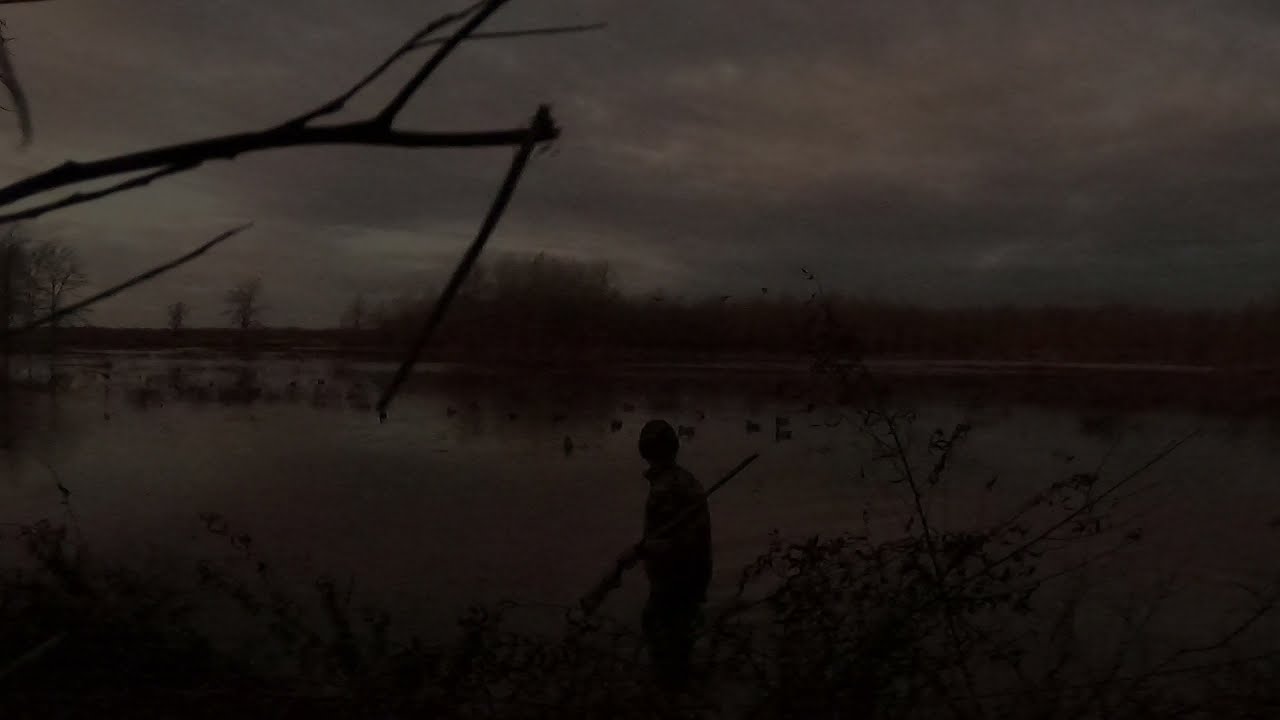The image presents a dark and moody scene that resembles a painting more than a photograph, largely due to its murky and shadowy atmosphere. The background features blackened skies, heavily clouded, evoking a sense of winter gloom. In the foreground, a man stands, perhaps knee-deep in water, clad in a camouflage coat with a hood obscuring his head, and holding a long shotgun. The dry, leafless trees and brush indicate a barren, winter landscape, likely a marsh or swampland. Despite the figure being largely in silhouette, his posture and the context suggest he is a middle-aged hunter. The presence of ducks in the water further supports this, depicting a scene of duck hunting amidst a desolate and almost eerie environment. The overall color palette is dominated by dark browns and grays, enhancing the somber and mysterious mood of the scene.